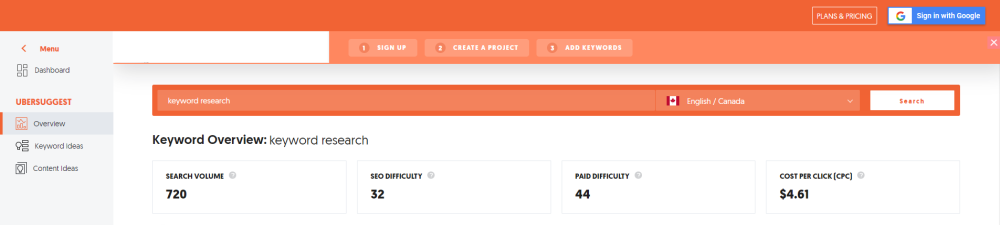This vibrant website features a header with a gradient background transitioning from an orangey-melon color on the left to the right. On the far right, it displays options like "Plans and Pricing" and a blue box reading "Sign in with Google." This blue box contains a white square with a prominent Google 'G' logo. To the left of this blue box is an area labeled "More," though the text following it is faded and difficult to read, possibly stating "card deep card" suggested by users, followed by small gray writing in a gray box.

The top navigation includes options to "Sign Up," "Create," and "Project." Although the text is notably small and somewhat unclear, additional options appear to be available. Directly below this navigation bar, there's a language and region selection area, indicated by "Keyword Search," with "English" and "Canada" mentioned, and an adjacent search bar on the right.

Beneath the search bar is a detailed keyword analytics section displaying various metrics for keyword research. These include "Keyword Overview," along with specific data such as "Keyword Search," achieving a "March Volume" of 720, a "SEO Difficulty" of 32, a "Paid Difficulty" of 44, and a "Cost Per Click" of $4.61.